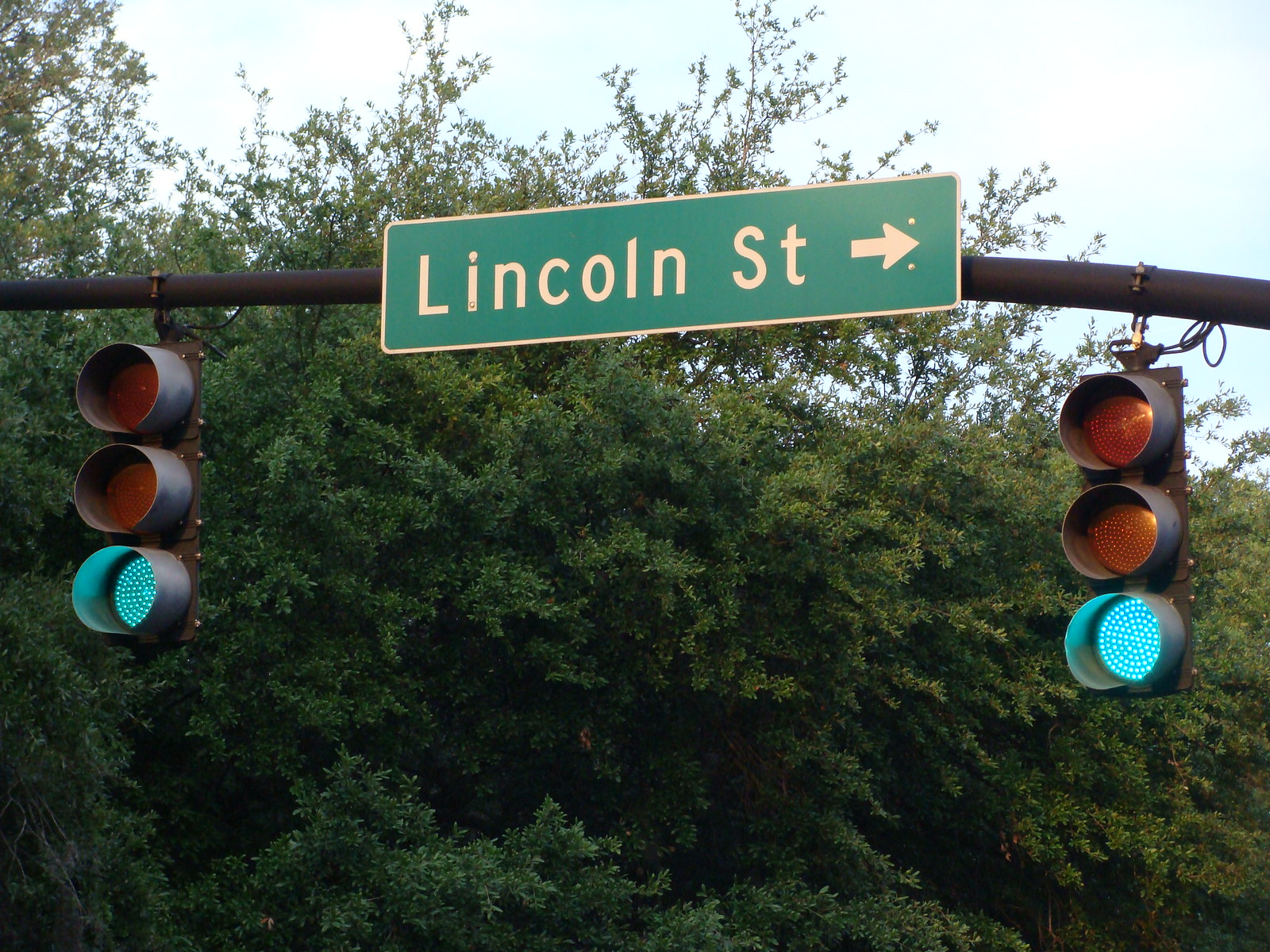The colour photograph, captured in landscape orientation, depicts an outdoor scene centered on a North American street sign and traffic lights. The rectangular street sign, with its green background and white perimeter, reads "Lincoln St" in slightly off-white letters, indicating Lincoln Street. The sign's distinctively curved edges frame a right-pointing arrow, and it's fastened to a horizontal metal pole by rivets—one on the dot of the 'i' and another at the bottom of the 'i,' as well as two more above and below the arrow's point. 

Suspended from either side of the pole are two traffic lights, each illuminated with a green light, the lowest of the three lights, signalling "go." The traffic lights, a very dark brown copper color, hang from the pole by visible wires. In the background, a dense grove of trees forms the primary backdrop, stretching across nearly the entire photo. These trees are lush and green, capped by a clear blue sky in the upper portion of the image, indicating a bright, cloudless day.